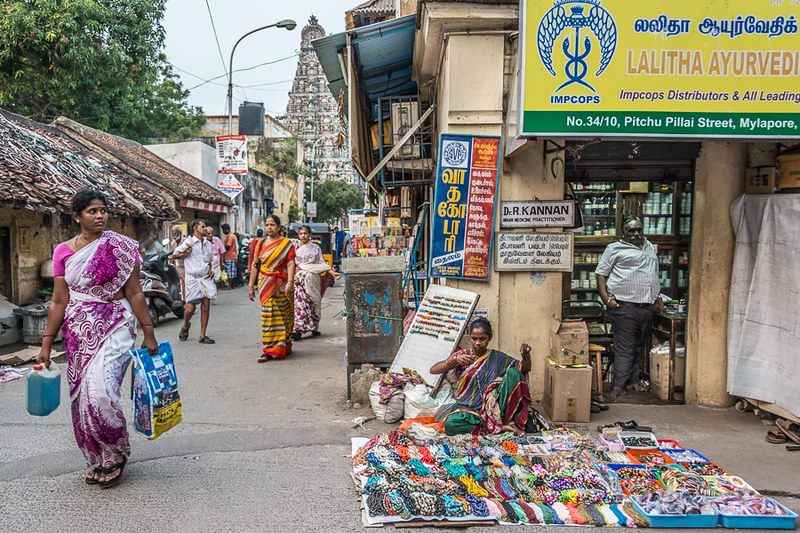In this vibrant photograph of an Indian street marketplace, the bustling scene captures numerous people, both men and women, strolling along a street lined with shops. The women, adorned in traditional saris, are seen carrying shopping bags and groceries. One vivid detail is a woman in the foreground dressed in a purplish-pink sari with white accents, balancing a blue bag and a large container of liquid. Nearby, a woman in orange and yellow attire contributes to the colorful atmosphere.

On the street's left side, a woman sits on the ground in front of a shop, meticulously displaying a variety of hand-made jewelry on a white mat. Her collection includes necklaces, bracelets, and other vibrant trinkets. Adjacent to her, inside the shop, stands a man who appears to be the storekeeper.

The street is lively with activity, featuring people engaged in shopping and conversation. A motorcycle is parked on the left side near a wooden structure, and a blue truck is visible further down the road. In the background, a tall, pyramid-shaped building with multiple levels looms against the skyline, partially obscured by tree leaves in the top left corner. This bustling marketplace scene authentically captures the essence of daily life in a small Indian town.